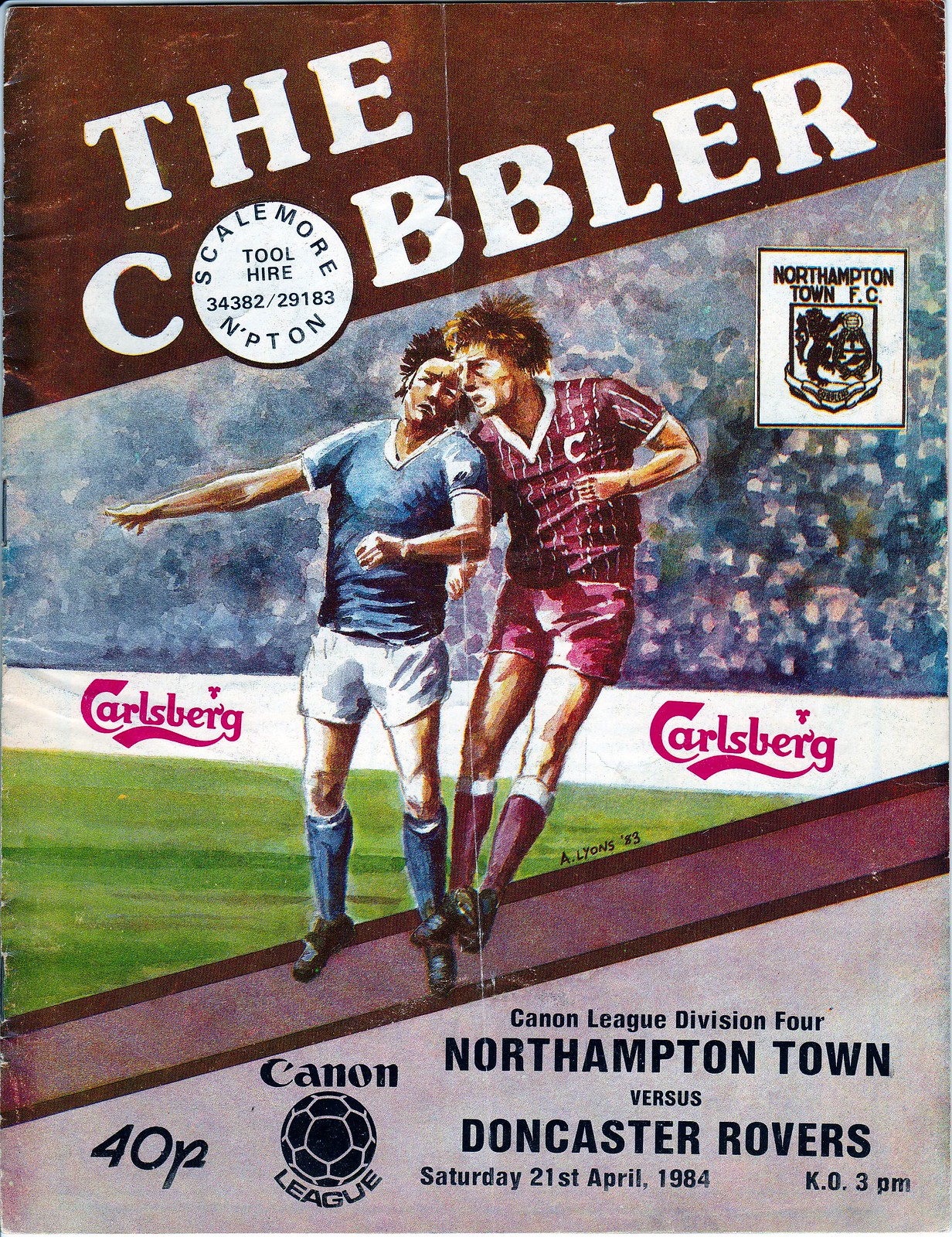The poster features a dramatic soccer match advertisement. At the top left corner, in bold white letters, it reads "The Cobbler," with additional content intricately inscribed within the letter 'O.' This content includes phrases like "Scale more, more ampton" and the numbers "34382/29183." Dominating the center of the image, two soccer players, depicted in action, are locked in a physical contest. The player on the left wears a blue jersey, white shorts, long blue socks, and shinguards, and is slightly shorter than his opponent. The opposing player is clad in a maroon jersey marked with a 'C,' matching maroon shorts, and reddish shinguards. This player is positioned to the right and appears taller. Behind them, a crowded soccer arena grandstand features a sponsor banner for Carlsberg. The right side of the image near the top also has the text "Northampton Town F.C." Finally, at the bottom right edge of the poster, in black letters, the event details are displayed: "Cannon League Division Four, Northampton Town vs. Doncaster Rovers, Saturday 21st April 1984, KO 3 PM." Adjacent to this text, an image of a soccer ball reinforces the competitive spirit of the match.